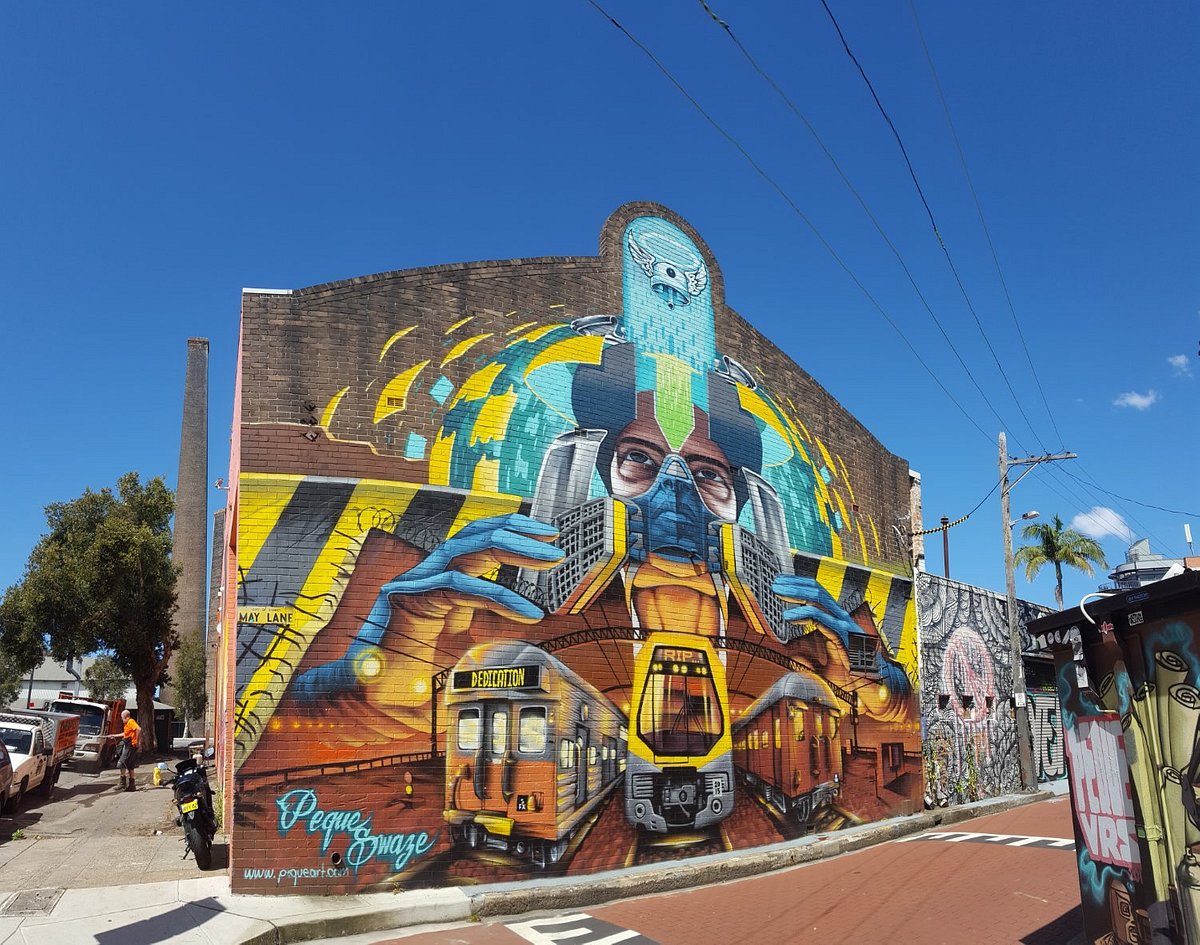The photo captures a vibrant and intricate street mural painted on the side of a brick building in a metropolitan area. The centerpiece of the mural is a sci-fi inspired figure whose body morphs into a train, embodying themes of urban life and movement. The figure, adorned with a blue headdress featuring a central skull, has expressive hands; one clutching a smaller train while the other seems to gesture outward. Above the figure's forehead, a helmet with angel wings floats almost like a halo, adding an ethereal touch. The mural is awash with bright and bold colors including yellows, blues, and reds, with an orange-tinted subway section depicted below the figure. Urban structures, trains, and tracks interweave throughout the artwork, emphasizing interconnectedness. In the foreground, stone or brick pathways and parked cars on the left add to the urban feel, while a logo with "PAKE SWAYS" and website information occupies the bottom left corner. The overall style is reminiscent of dynamic graffiti art, rich with depth and complexity through added images and patterns in the background.